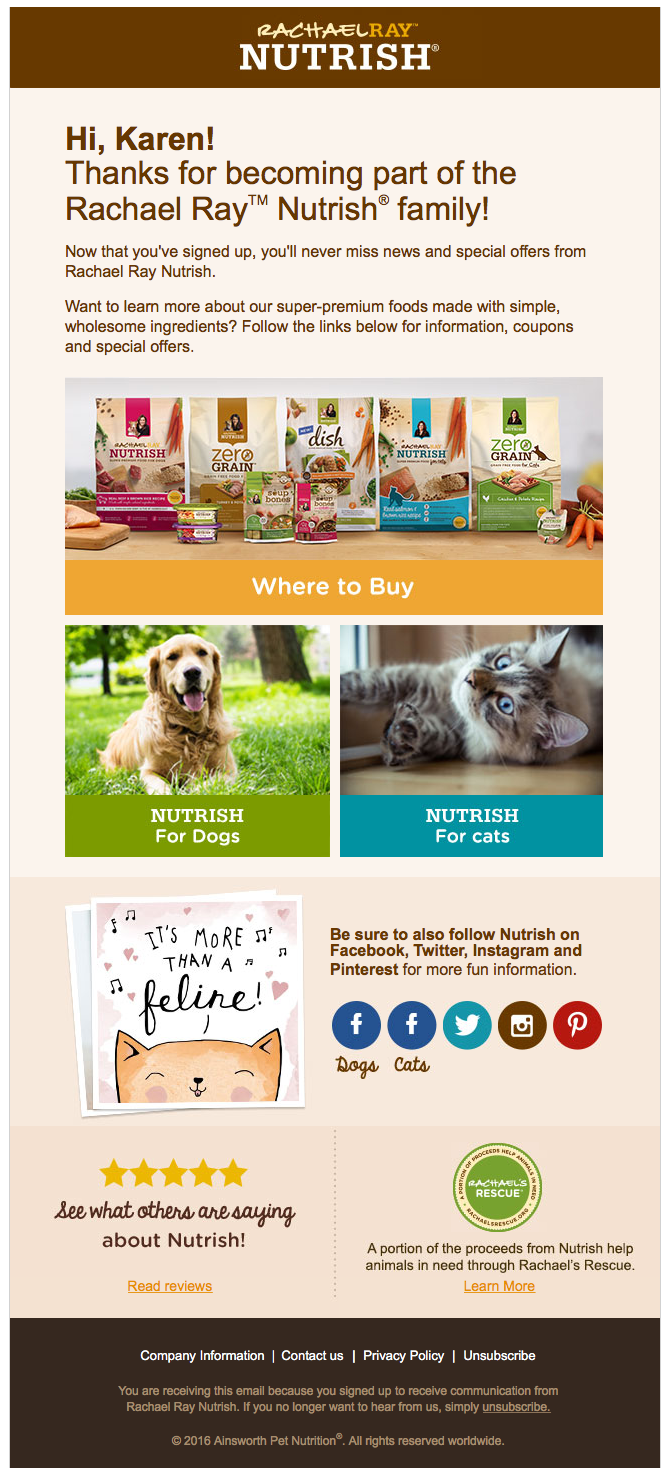In this promotional image, we see celebrity chef Rachael Ray introducing a new member to the Rachael Ray Nutrish family. The image welcomes Karen for becoming part of the Rachael Ray Nutrish registered community. It ensures that, as a registered member, Karen will receive the latest news and special offers from Rachael Ray Nutrish. The image invites the viewer to learn more about Rachael Ray’s super premium pet foods, made with simple and wholesome ingredients. The message encourages Karen to follow the provided links for information, coupons, and special offers, highlighting categories such as Zero Grain, Nutrish Dish, Where to Buy, Nutrish for Dogs, and Nutrish for Cats. Testimonials and reviews are available for pet owners to see what others are saying about Nutrish. The caption also encourages viewers to follow Rachael Ray Nutrish on social media platforms like Facebook, Twitter, Instagram, and Pinterest to stay updated with more fun information and links related to pet care and products.